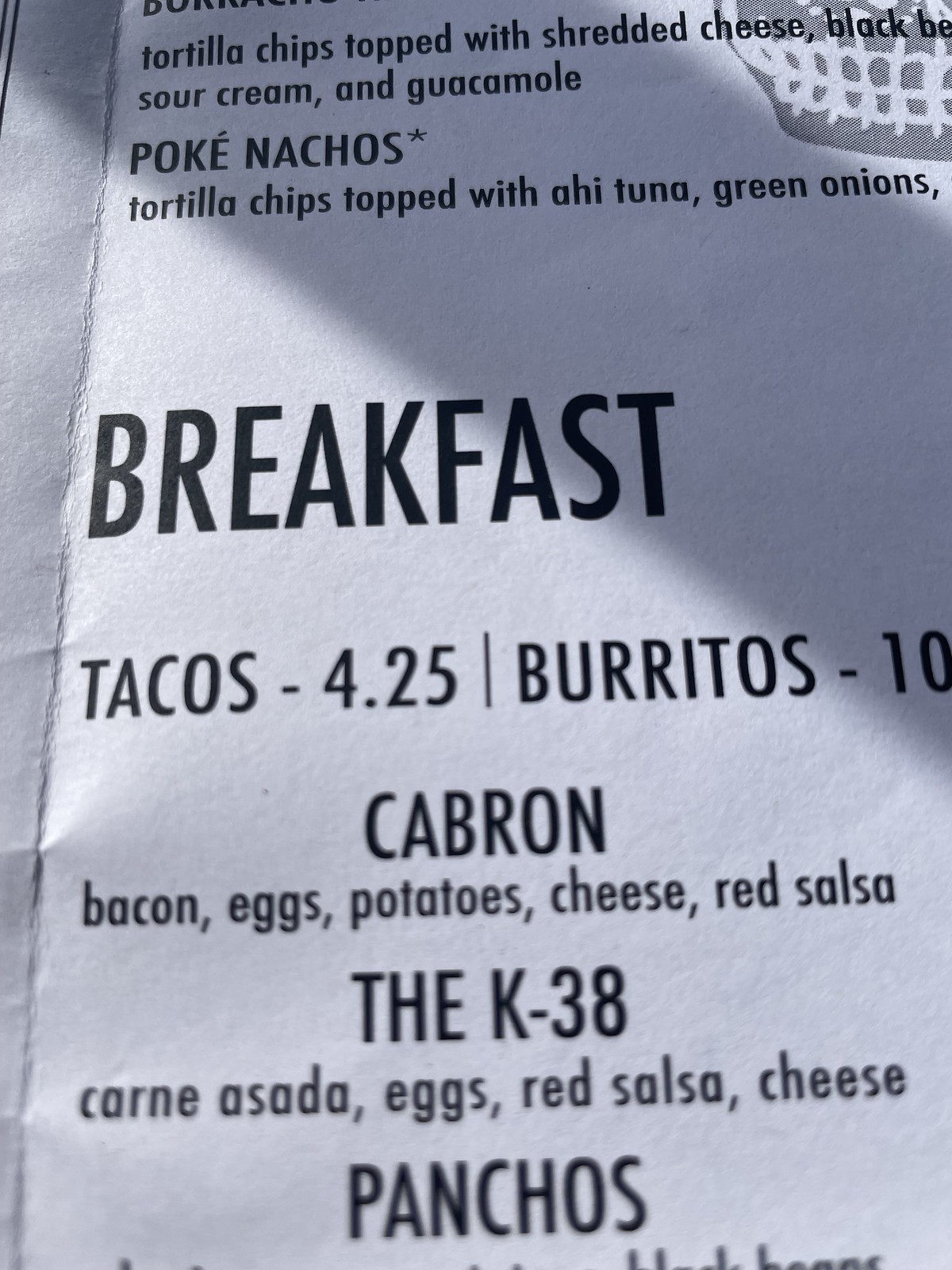The image depicts a close-up of a creased paper menu with black text on a white background. At the top, the menu lists "Tortilla chips topped with shredded cheese, black beans, sour cream, and guacamole." Below that in larger letters, it reads "Pokey Nachos," followed by "Tortilla chips topped with aji tuna and green onions." The next section is labeled "Breakfast." Under this heading, it includes "Tacos - $4.25," "Burritos - $10," and an item named "Cabron," described as containing "Bacon, eggs, potatoes, cheese, and red salsa." Further down, in larger print, is "The K-38," which includes "Carne asada, eggs, red salsa, and cheese." The final listed item, also in large letters, is "Ponchos," but the description is cut off. The menu has noticeable creases from being folded and a diagonal shadow obscures the top half of the picture.